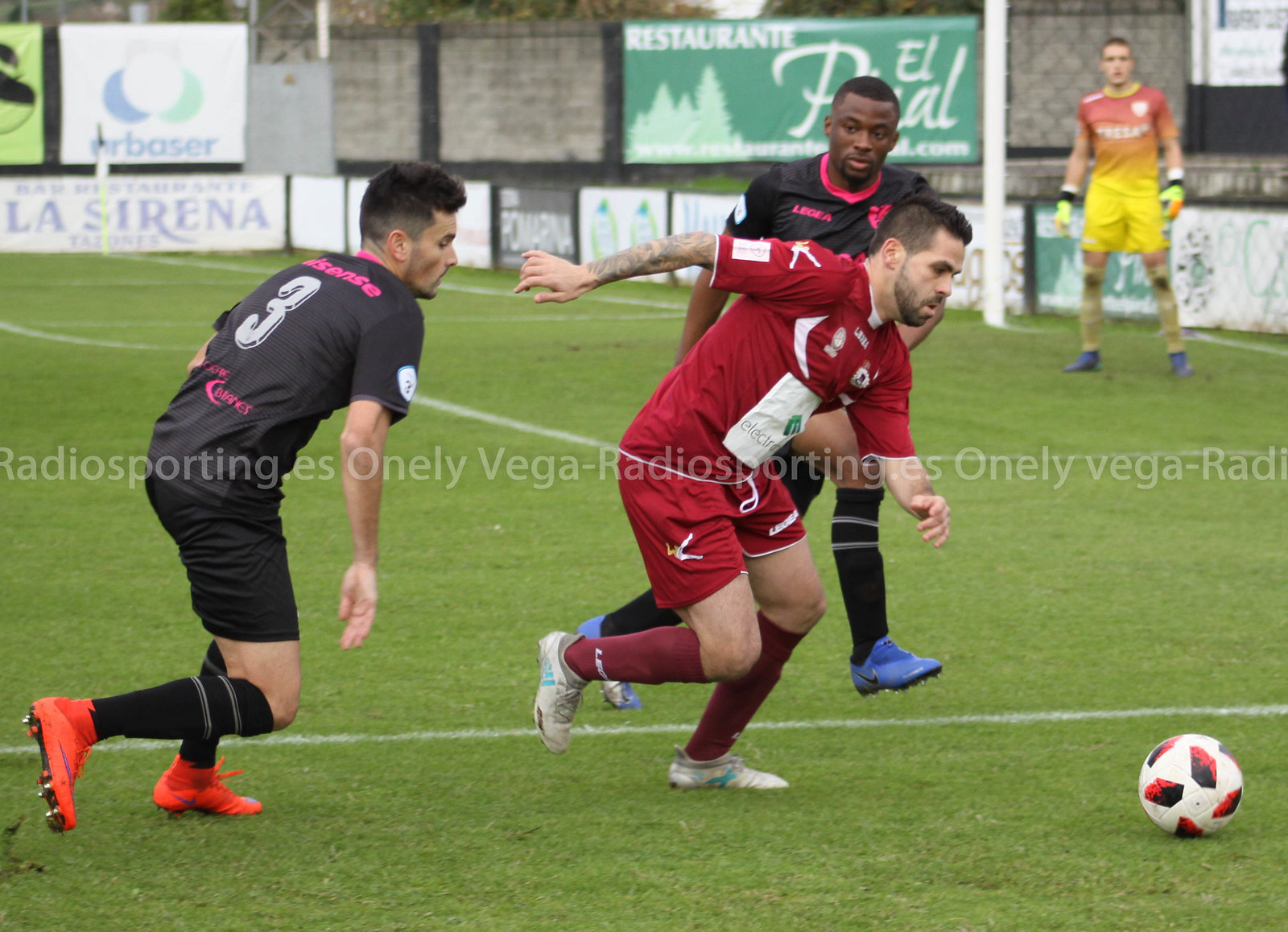The photograph features a dynamic soccer match between two teams on a lush, green outdoor soccer field marked with white lines. The focus is on a player in red and white attire—red shirt, shorts, and socks with white accents—preparing to kick a black, white, and red soccer ball. Surrounding this player are two opponents dressed in primarily black uniforms, which include subtle white elements and pink writing. In the background, a goal is visible in the top right corner, characterized by its square-shaped metal frame and black netting. Stationed in front of the goal is a goalie, distinguished by his bright yellow gloves, long yellow shin guards, yellow shorts, blue shoes, and a red and yellow shirt, ready to defend. The image beautifully captures the intensity and color of the game.